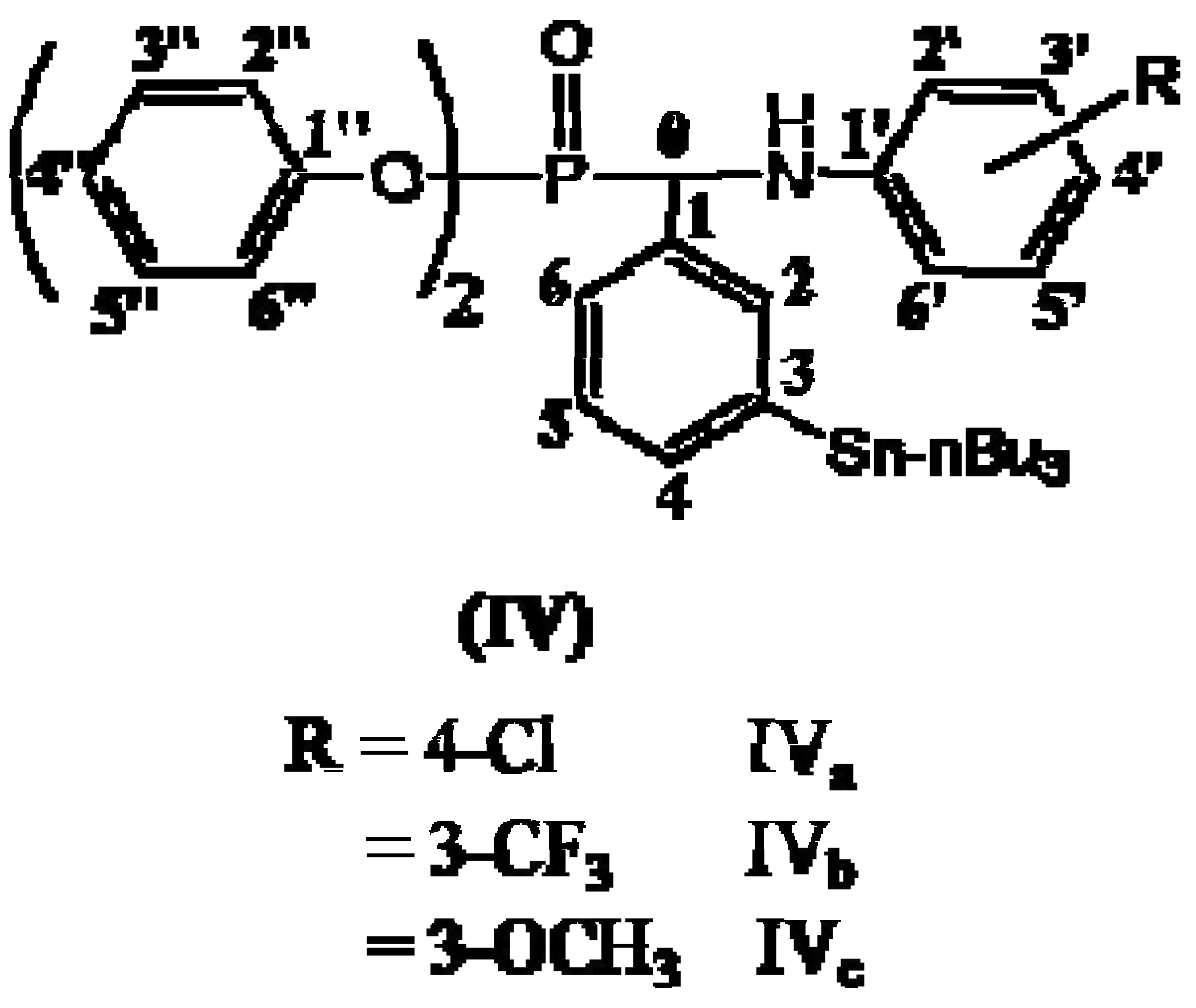This image depicts a detailed molecular structure of a chemical compound. The structure includes three six-sided hexagonal rings, each point of the hexagon labeled with numbers. Starting with the first hexagon from the middle left point and moving clockwise, the points are labeled with 4', 3', 2', 1', 6', and 5'. This hexagon is enclosed in parentheses with a subscript '2' below the parentheses. A single line connects it to an oxygen (O) atom, which is then connected to a phosphorus (P) atom by a single line and a double line to another oxygen (O) atom. Another single line connects the phosphorus atom to a second hexagon, similarly numbered, which is followed by a string of letters: S-N-n-BUG.

To the main horizontal line of the formula, the letters H, N lead into the third hexagon. Starting again from the middle left point and moving clockwise, the points are labeled 1'', 2'', 3'', 4'', 5'', and 6''. A line goes from the center of this hexagon to the letter R on the outside of the hexagon. Below this structural diagram is a guide specifying different values for R: '(IV)' followed by 'R = 4-Cl, IVa', '= 3-CF3, IVb', and '= 3-OCH3, IVc'. The chemical notation is complex and pixelated in parts, making it challenging to read but providing a comprehensive depiction of the compound's molecular structure.